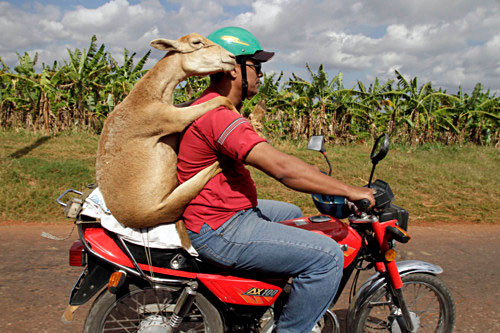In this captivating photograph, a tan male is seen riding a smaller, red motorbike adorned with black and silver accents, and equipped with two rearview mirrors. The rider sports a teal helmet with a gold decal and is dressed in a red short-sleeve shirt paired with blue jeans. What makes this image truly unique is the sheep perched on the passenger seat behind him, seated in an almost human-like manner. The sheep steadies itself with its front hooves placed on the rider's shoulders and its back hooves around the man's chest. It rests on a blanket that appears securely fastened to the bike.

The scene unfolds on an asphalt road bordered by lush green grass. In the background, a variety of tropical-looking bushes and distant trees create a serene, natural setting under a bright blue sky dotted with fluffy white clouds. The overall composition of the photograph captures an extraordinary moment of companionship and gentle adventure against a picturesque, tropical landscape.